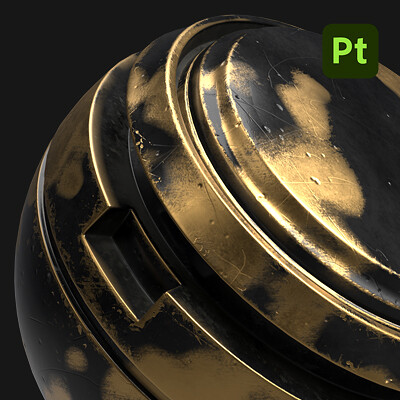The photograph is a close-up of a metallic object that appears to be brass or perhaps a black material spray-painted with gold. The object is round with a worn, tarnished appearance, revealing black discoloration in several areas. It might resemble parts of a doorknob or a round lock, with a circular top and an attached but separate bottom piece. A rectangular indent is centrally positioned on the object. The background of the image is black, and in the upper right corner, there is a dark green square with light green letters that say "P" and "T," with the "P" being capitalized and the "T" in lowercase. The photo is taken at a diagonal angle, emphasizing the worn texture and the intricate assembly of the metallic object.